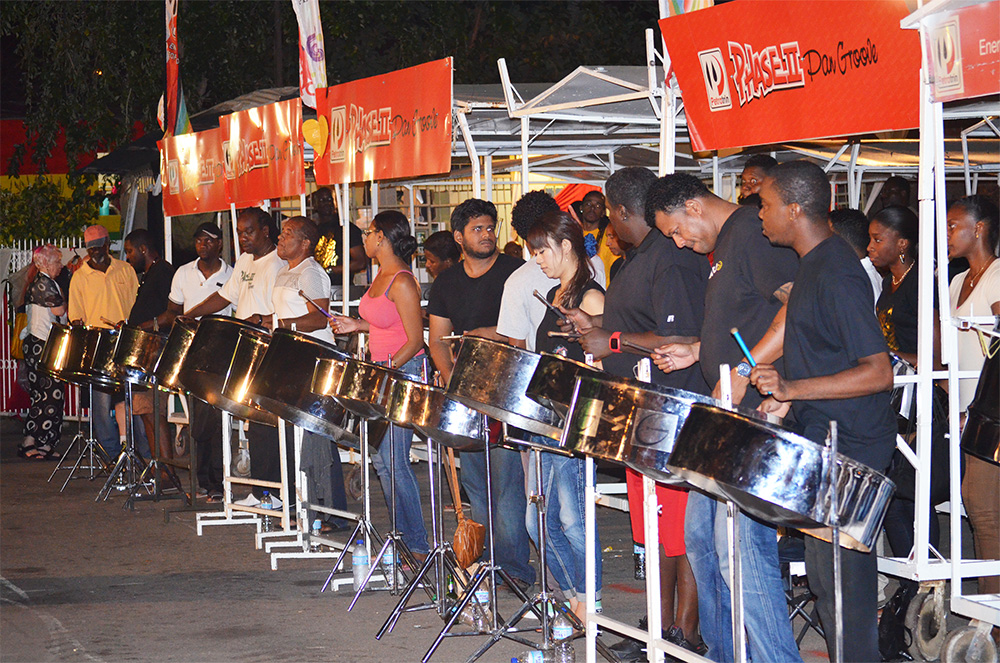In this nighttime photograph, a diverse group of men and women are participating in a vibrant drumline performance, set against a dark sky that contrasts with the illuminated scene below. The setting appears to be an outdoor parking lot or street, surrounded by a patchwork of makeshift structures and green foliage visible in the background, alongside a white picket fence. The drumline consists of nine shimmering metal drums, each of varying sizes but all reflecting light brightly. Lined up from left to right, we see three African American men in white shirts, a woman in a pink shirt, a presumed Spanish man in a blue shirt, an Asian woman, and three more African American men, all focused on their instruments.

Above the performers, a canopy supports a series of large red banners, one of which reads "Phase Two," though further text is difficult to decipher. These banners hint at a festival or competition context, inferred also from the crowd of onlookers gathered behind the players. The audience adds to the communal atmosphere of the event, emphasizing the shared cultural experience. The scene is rich with the promise of synchronized beats and communal celebration, highlighted by the mixed-race participation and the vivid array of colorful attire.